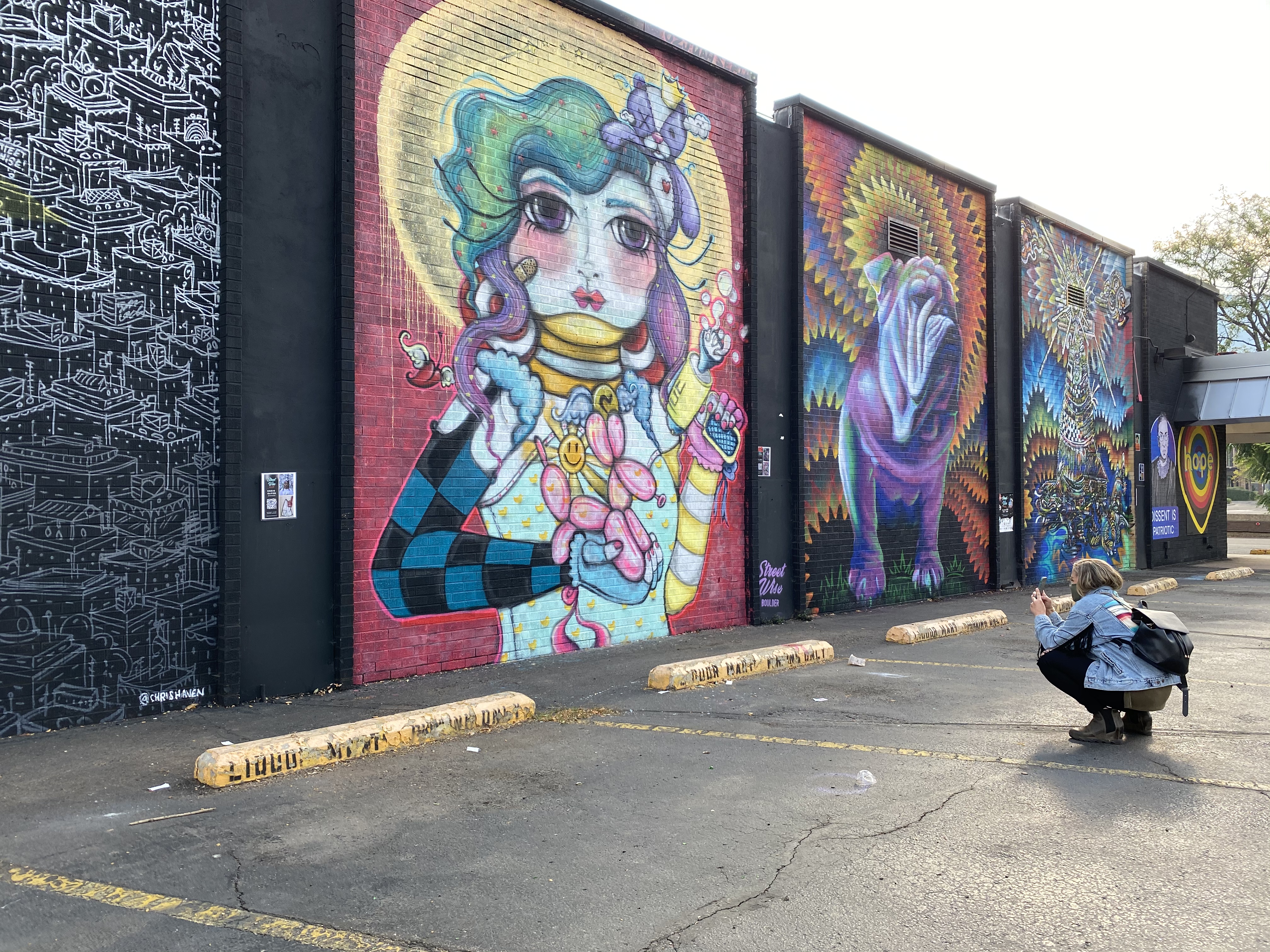This photograph depicts a vibrant graffiti mural spanning the length of a battered parking lot wall, divided into five distinct panels, each corresponding to a parking space. The parking lot itself features cracked black asphalt and aging yellow paint marking the parking spots and bump stops.

Starting from the left, the first panel showcases a dense urban scene on a black background with white outlines illustrating buildings stacked atop one another. The second panel features a striking image of a girl with green tentacle-like hair, wearing a blue and yellow shirt with a blue and black checkered sleeve. She holds a balloon animal of a dog in her right hand and a bubble gun in her left, with a stuffed animal peeking from the top right of the image.

The third panel portrays a purple mythical creature resembling a dog, surrounded by swirling waves of orange and yellow light, and standing on green grass. The fourth panel is a detailed depiction of a tower with a firework explosion at the top, set against a blue background that may represent water, with accompanying elements surrounding the scene.

The final panel on the far right features a circular design with black, yellow, and orange hues, encapsulating the word "HOPE" in bold yellow text.

Additionally, a woman is seen kneeling in the parking lot, taking pictures of the striking mural, further emphasizing the captivating nature of this vibrant streetside art.